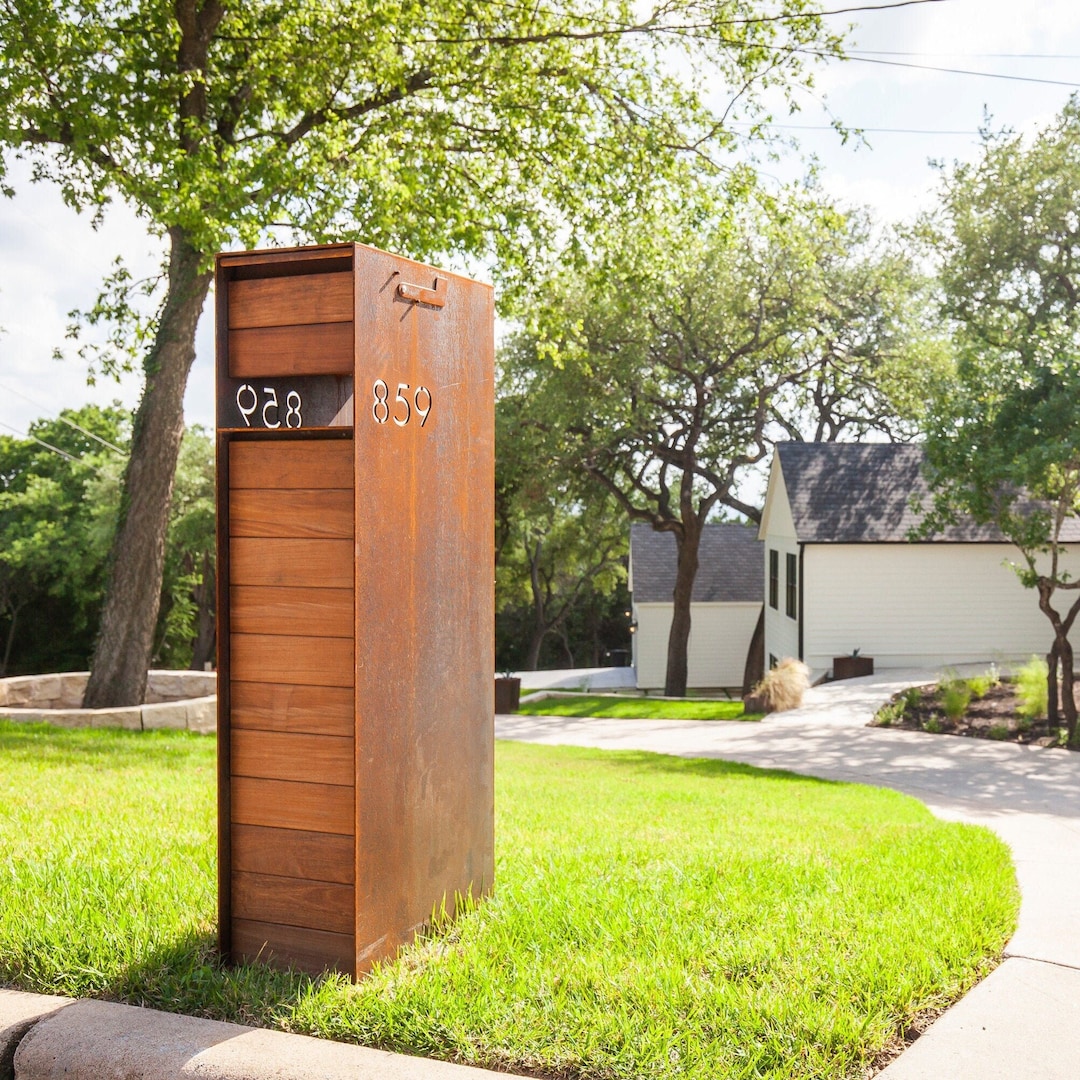This photograph captures a modern-style, narrow, rectangular mailbox standing prominently in the front left-hand side of a grassy, circular lawn near a concrete curb. The mailbox, made of cedar wood slats, features engraved house numbers "859" on both sides, accompanied by a flag positioned above the numbers. The mailbox extends all the way to the ground, designed to receive packages easily. In the background, to the left, a tree leans slightly to the right, with a visually engaging masonry work around its base. The yard, with its winding pathway and lush greenery, includes various other trees and bushes. The pathway meanders beside the mailbox, leading towards a large, white house with a dark roof and two dark windows visible. The house, appearing expansive, sits behind this picturesque yard, complementing the residential area's aesthetic charm. There is also an indication of additional structures like a garage or outbuilding adjacent to the house. The edge of the street and a significant amount of cement work frame the scene, highlighting the neat, modern curb appeal of this suburban setting.